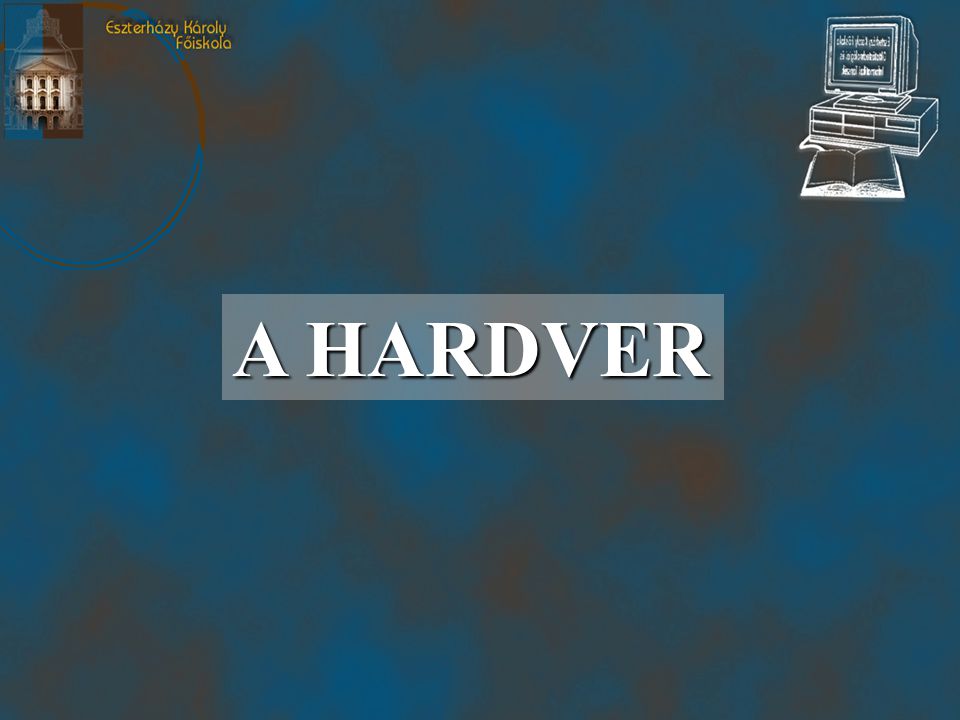The blue poster features a central focus on the phrase "A HARDVER" in white text. The background, a smoky blue, gives the appearance of swirling smoke. In the upper left corner, there is an artistic rendering of an elegant, old building accompanied by the text "ESZTERHAZY KAROLY FOISKO" in small golden letters, suggesting an Eastern European origin. The upper right corner displays a sketched image of an outdated computer with a large monitor and a book placed in front of it.